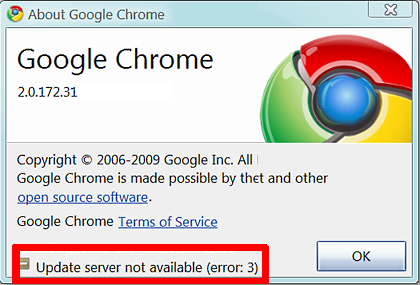Detailed Caption:

A screenshot displaying the "About" window in Google Chrome is shown. In the upper left-hand corner of the window, a small dialog box is visible. The focal point of the image is the Google Chrome logo, followed by text indicating the browser's version number: 2.0.172.31. Below this, a line of text notes the contribution of Thet (spelled out as T-H-E-T) and other open-source software to the development of Google Chrome, dated from 2006-2009. Additionally, the Google Chrome Terms of Service is presented as a clickable link for more information. Towards the bottom of the window, a message circled in red draws attention to an error notification stating "Update Server Not Available, Error 3." Adjacent to this error message is an "OK" button that can be selected.